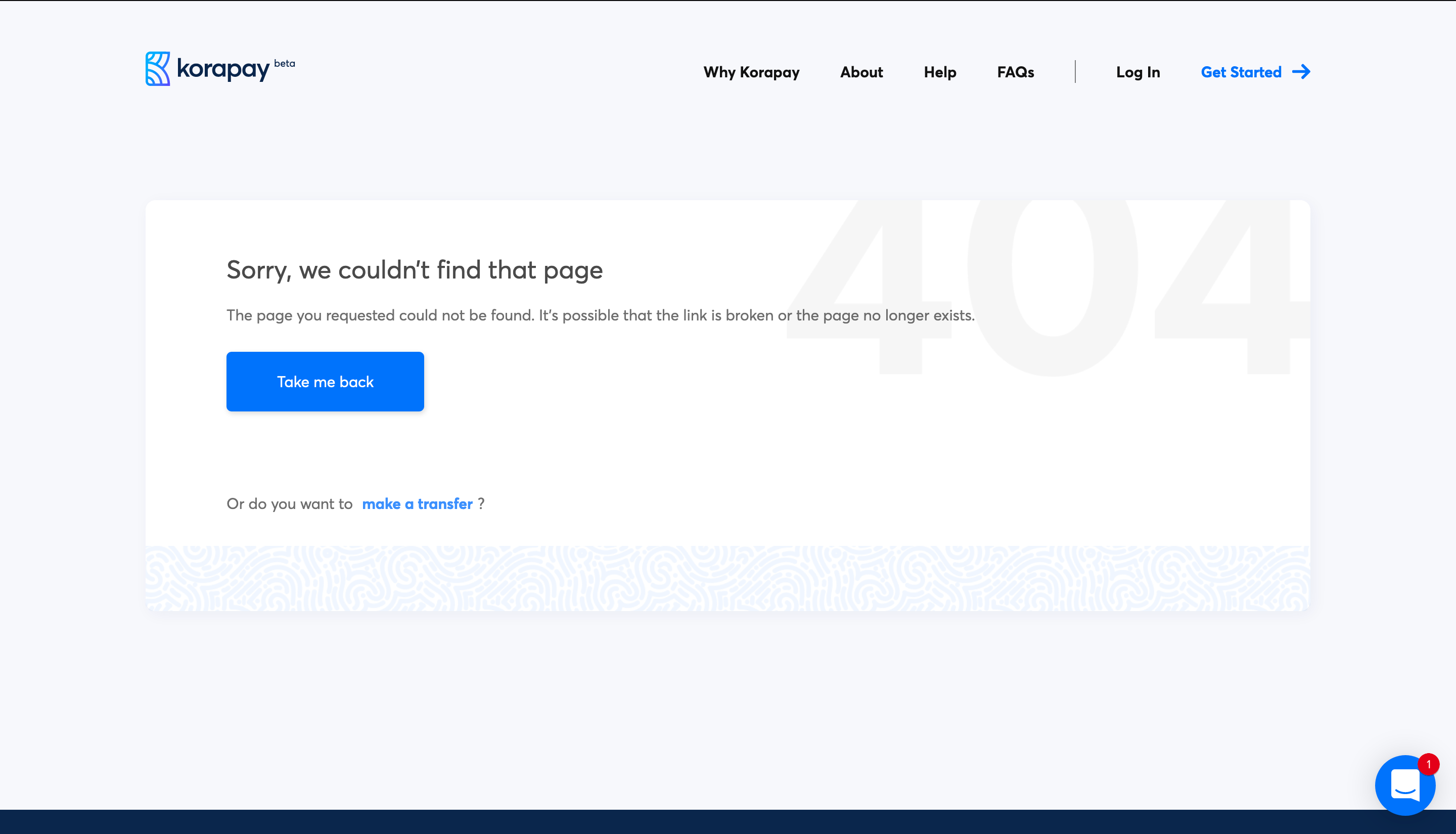**Descriptive Caption:**

The image portrays a Coropay webpage with a light grey background. At the top left corner of the screen, the Coropay name and logo are prominently displayed. Opposite to the logo, horizontal menu headings read "Why Coropay," "About," "Help," and "FAQs." Dividing the main menu from the secondary actions is a fine grey bar, followed by additional headings "Login" and "Get Started," with "Get Started" highlighted in blue and an accompanying blue arrow pointing to the right.

Centrally placed on the screen is a large white rectangle, displaying a prominent "404 Error" message. The dialogue box states, "Sorry, we couldn't find that page. The page you requested could not be found. It's possible that the link is broken, or the page no longer exists." Below this message is a blue button labeled "Take me back." Beneath the button, an additional line of text asks, "Or do you want to make a transfer?" with the phrase "make a transfer" highlighted in blue.

At the very bottom of the screen runs a fine dark blue line. Positioned in the bottom right corner is a circular chat window icon, marked with a red notification badge indicating "1" new message.